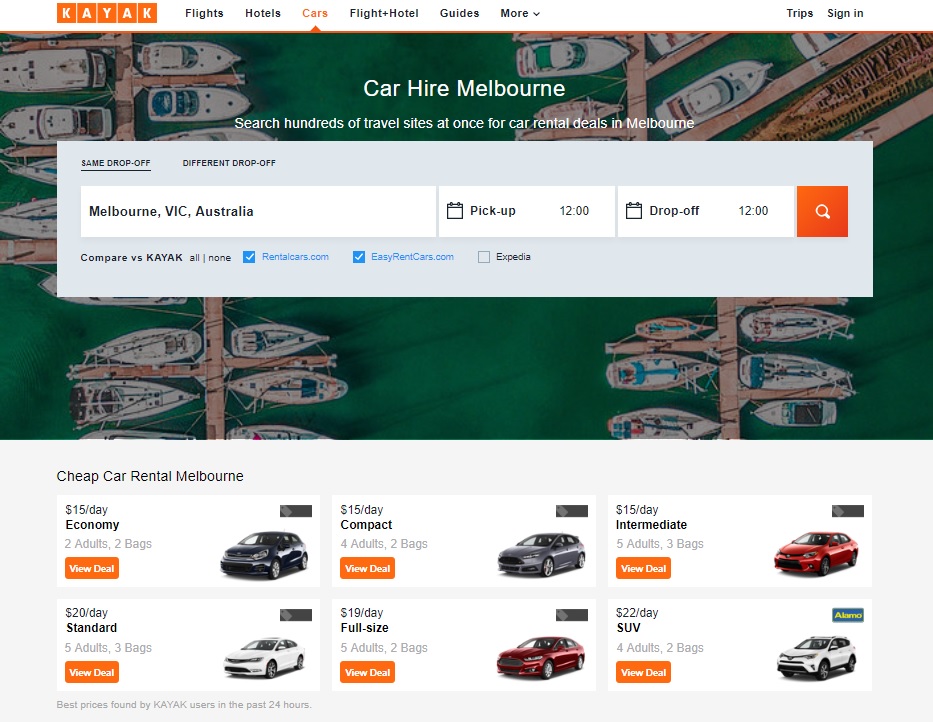The website displayed is Kayak, recognizable by its logo positioned in the upper left corner within orange boxes and white letters. Adjacent navigation options include 'Flights,' 'Hotel,' 'Car,' 'Flight + Hotel,' 'Guides,' and a 'More' dropdown menu. In the top-right corner, options for 'Trips' and 'Sign In' are present. 

The webpage features an aerial photograph of a marina with numerous ships and boats docked. Superimposed on the image in white text is the header: "Compare Car Hire, Melbourne." The text prompts users to "search hundreds of travel sites at once for car rental deals in Melbourne."

Below this, a grey rectangular box presents user options for car rental search criteria. Two tabs are present: 'Same Drop-off' and 'Different Drop-off,' with 'Same Drop-off' being the selected option. The location is set to "Melbourne, Vic, Australia," with a pickup and drop-off time at 12:00 PM. The search button is prominently displayed in an orangey-red color beneath these options.

Further down, a section gives options to compare Kayak with other sites such as 'Compare vs. Kayak,' 'RentalCars.com,' 'EasyRentCars.com' (both ticked), and 'Expedia' (not ticked). 

The bottom section shows a grid of cars featuring three cars per row and two rows in total. The heading reads, "Cheap Car Rental Melbourne," with a starting price of $15 per day for economy cars.